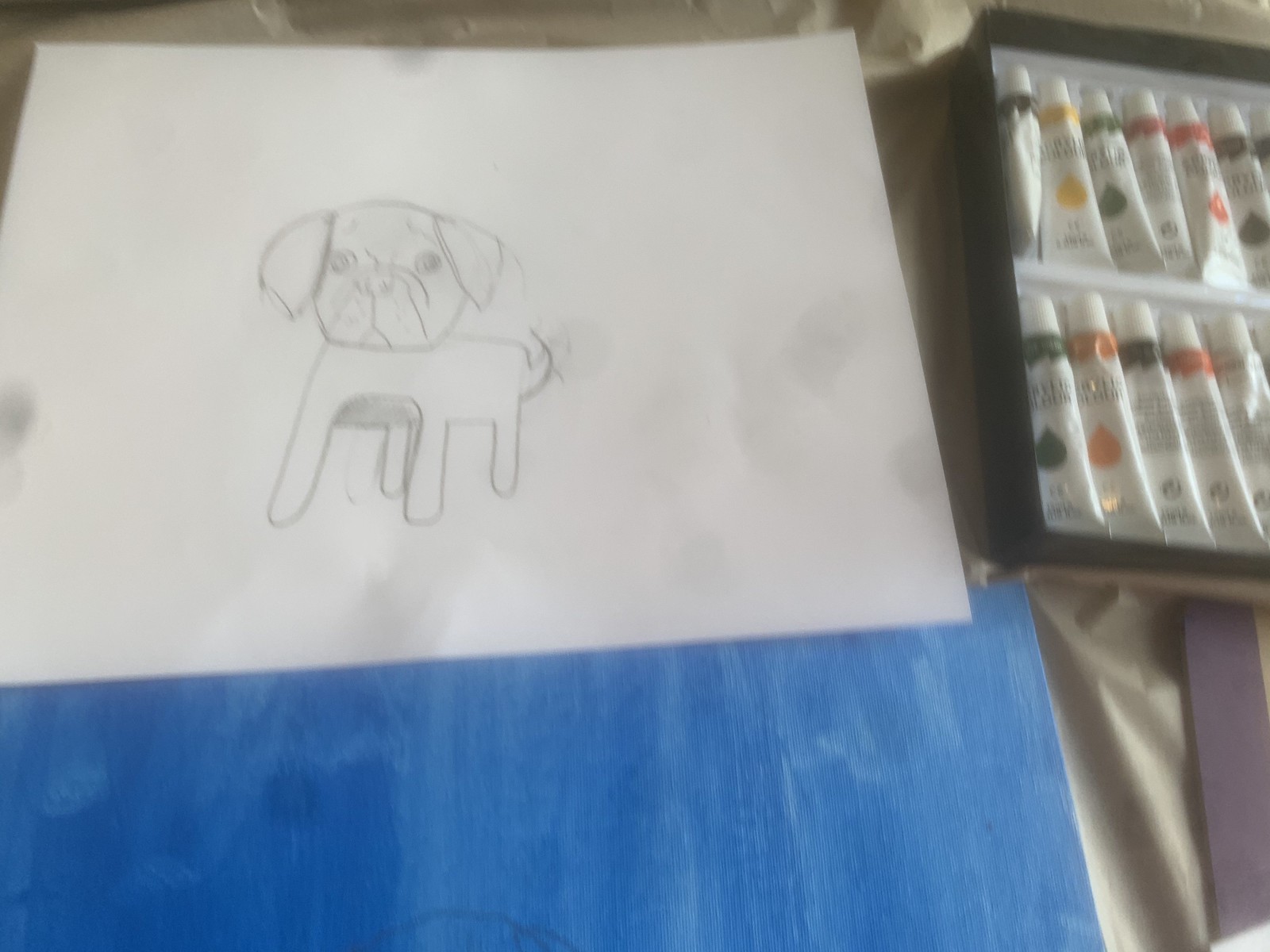In this detailed photograph, a white sheet of printer paper displays a pencil drawing of a dog, characterized by its floppy ears, rounded eyes with a glowing effect, nose, mouth, and a squarish body with all four legs visible. The dog's tail is pointed up, and it appears to be looking off into the distance. The drawing style is simple, with visible pencil marks and evidence of erasure, suggesting it might have been created by a younger artist. Beneath the drawing lies a blue canvas or piece of painted wood. To the right side of the image, various tubes of acrylic paint are partially visible within a box, showcasing a range of colors including reds, greens, yellows, blacks, and ochres. The entire setup is placed on what appears to be a cloth or tablecloth, creating a first-person point-of-view composition in a horizontal landscape format.